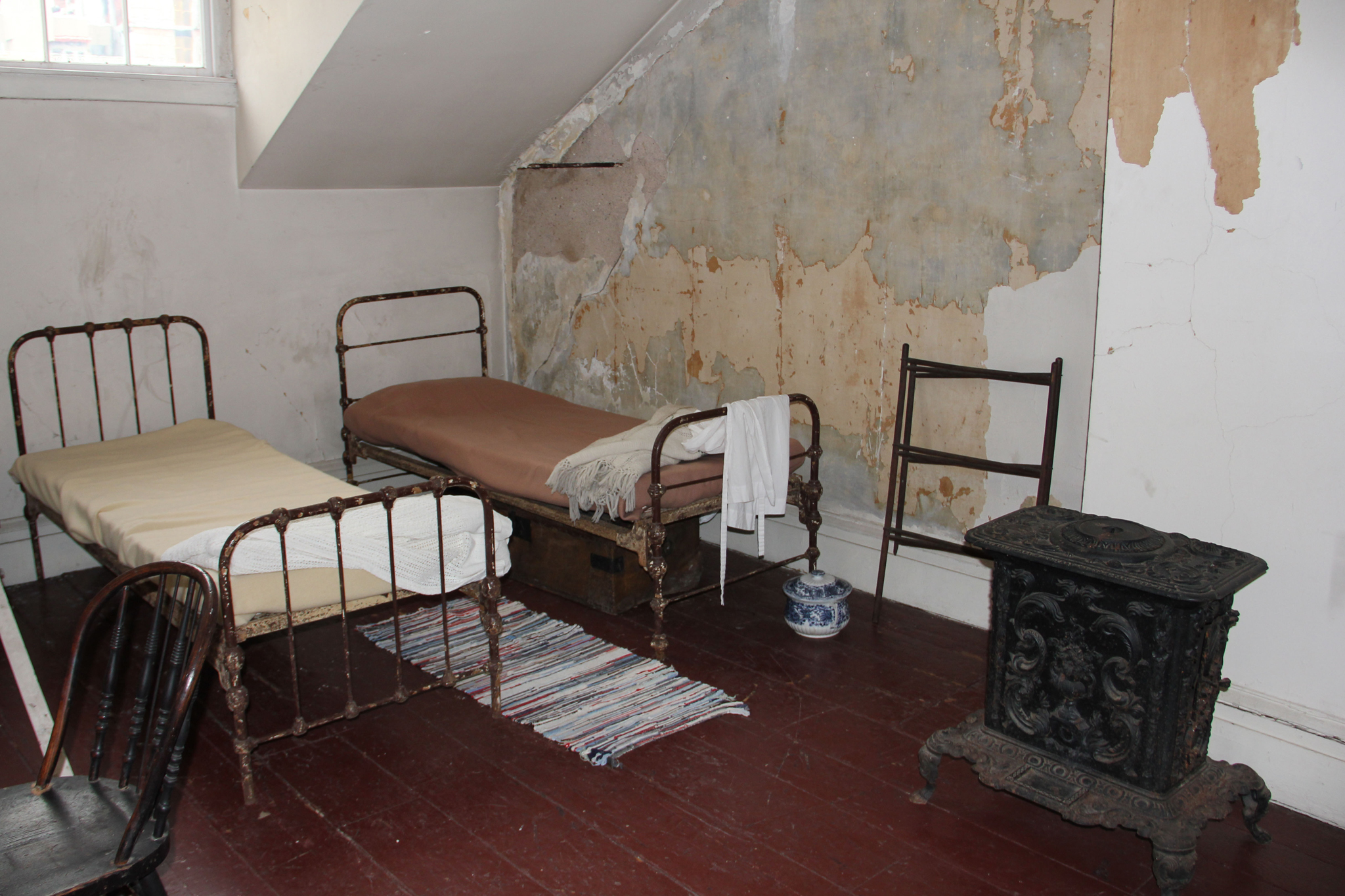The image depicts a dilapidated room dating back to around 1900, evocative of a servant's quarters. The walls, painted in a now-faded cream color, show signs of neglect with areas where the paint has peeled off. Two very old, thin iron beds dominate the space, their metal frames darkened with age. One bed is covered with a white sheet, while the other sports a brown blanket. A homemade round rug lies between the beds, and underneath one bed, there's an old trunk. A chamber pot can be seen beside one of the beds, enhancing the historical authenticity of the scene. Above one of the beds, a small window allows minimal light to filter in. To the side, a dark wooden chair and a small black nightstand provide sparse furnishings. A folding frame for clothing stands nearby, adding to the room's utilitarian atmosphere. The floor is dark wooden floorboard, completing the picture of a modest, timeworn dwelling likely belonging to domestic servants from the early 20th century.